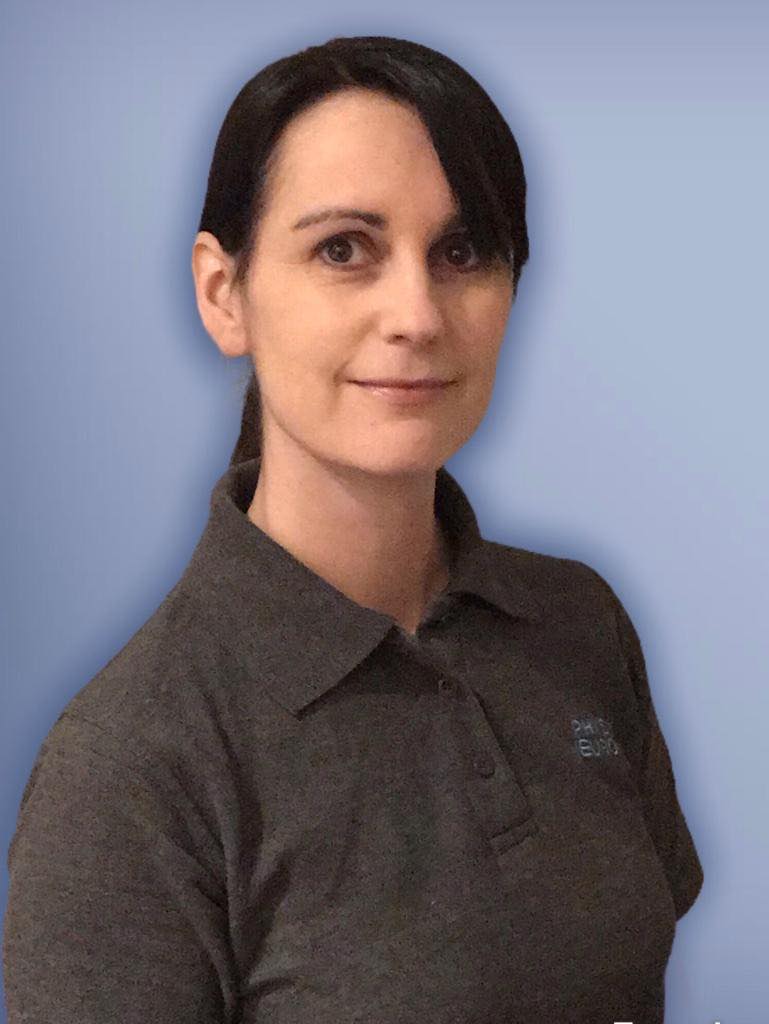This image is a detailed color portrait of a young woman, appearing to be in her 30s, standing against a light blue backdrop with a faint artificial shadow effect around the image. She has long black hair, styled with bangs that sweep from her left eye toward her left ear, while the right side of her face has no bangs, revealing her left ear and possibly a ponytail behind her. She has brown eyes and a slight half-smile on her face. She faces the camera, but her body is angled slightly with her left shoulder pointing away. She is wearing a dark gray polo shirt with a collar and a partially unbuttoned top. There is an unidentifiable emblem on the left chest of the shirt, with the letters PH and B somewhat discernible, and a small, difficult-to-read name stitched in white on the right side. She is a Caucasian woman.